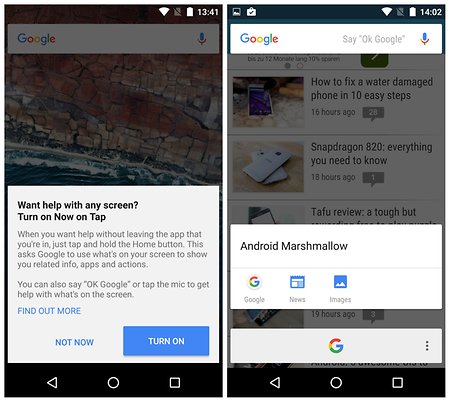This is a combined image of two separate screenshots, displayed side-by-side, from a mobile device.

On the left side, the screenshot features a dark, shadowed background with a faint image of a cliff with visible cracks, possibly with water beneath it. In the foreground, there is a prominent white dialog box that reads: "Won't help with any screen. Turn on now, on tap. When you want help without leaving the app that you're in, just tap and hold the Home button. This asks Google to use what's on your screen to show you related info, apps, and action." Below this message, two options are available: "Not now" on the left and "Turn on" on the right.

On the right side, the screenshot displays a Google search interface. At the top is the Google search bar, and at the bottom, there is a white box that reads "Android Marshmallow." In the background are faintly visible search results including "How to fix a water-damaged phone in 10 easy steps," "Snapdragon 820," and "Everything you need to know." At the very bottom of the screen, a white search navigation bar stretches across, featuring the Google icon (G) in its center.